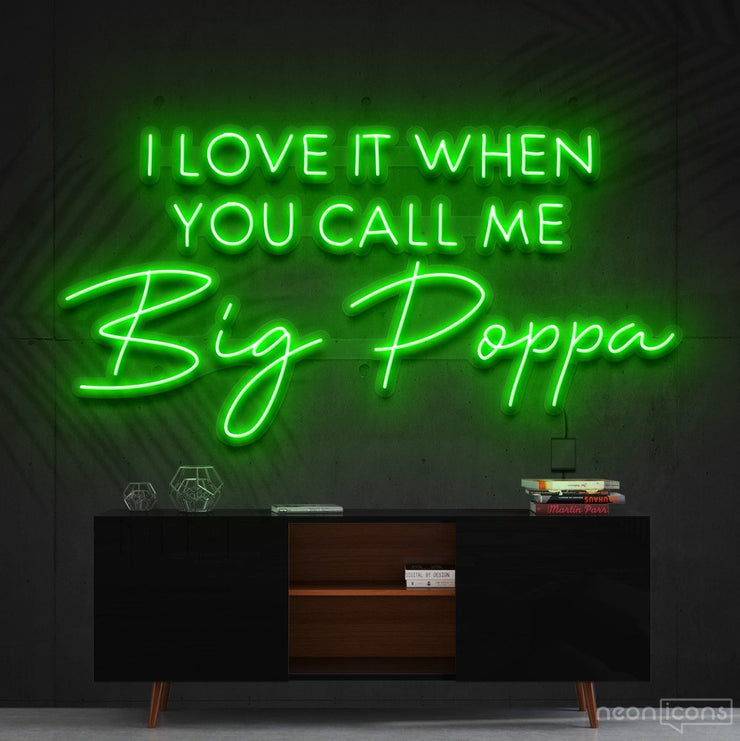The image likely depicts a digitally generated scene or an animation of a room with a focal point being a large, neon green sign on a dark gray wall that reads: "I LOVE IT WHEN YOU CALL ME" in uppercase letters, followed by "Big Papa" in cursive. The background wall features shadows resembling palm fronds. Below the sign is a sleek, black modern cabinet or bookshelf with brown legs and a wooden interior. On top of the cabinet, to the right, there's a stack of three books, and to the left, several geometric silver cubes and another book. The open middle section of the cabinet displays two white books.